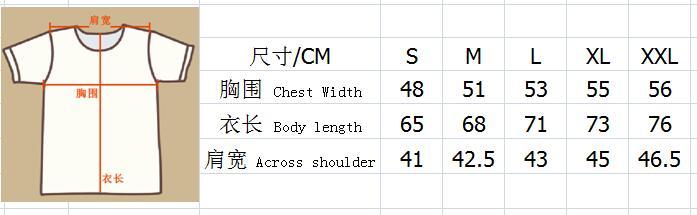The image is a detailed guide on how to measure for clothing sizes. On the left, it features a white t-shirt, outlined in black against a tan/brown background, with red lines indicating measurement points. To the right, there is a black and white grid displaying measurements in both Chinese and English. The grid lists measurements for chest width, body length, and across shoulder in centimeters for different sizes: small, medium, large, extra-large, and extra extra-large. For instance, a small size has a chest width of 48 cm, a body length of 65 cm, and an across shoulder measurement of 41 cm. The measurements increase incrementally for each subsequent size, with the extra extra-large measuring 56 cm in chest width, 76 cm in body length, and 46.5 cm across the shoulders.